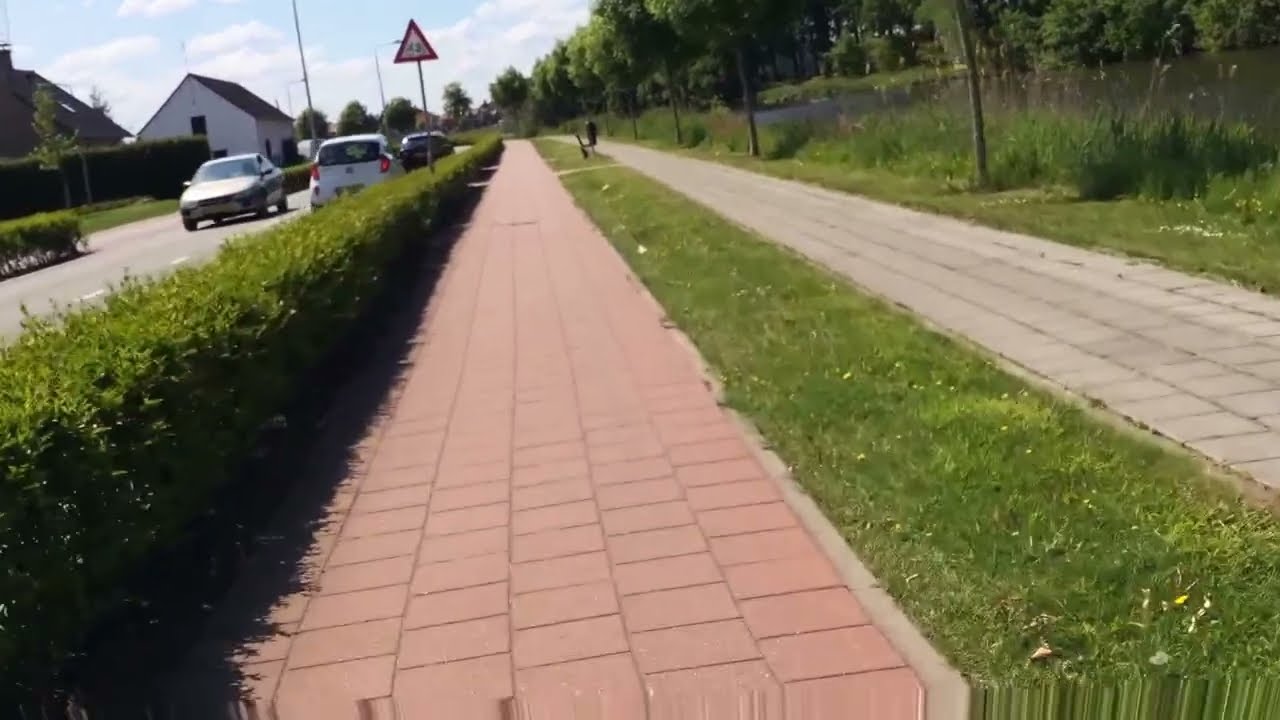This photograph, taken outdoors during the daytime, captures a structured and scenic environment. Dominating the center, a footpath made of pink-red bricks extends from the bottom to the top of the image. To the right of this path, a strip of neatly mowed green grass separates it from a secondary, slightly lighter grey footpath. Beyond the second pathway, a grassy expanse stretches towards a water body, flanked by trees and dotted with electrical poles. On the left of the central footpath, there is a well-maintained row of green hedges. Adjacent to these hedges is a two-lane road with white dashed lines, carrying vehicles both away from and towards the viewer. Further to the left, past the roadway, several houses are visible, set against a backdrop of a blue sky accented with white clouds. Additionally, there is a triangular road sign with a red border and white center, positioned at the top of the page, whose specific symbol is obscured. The vivid colors in the image include shades of red, green, grey, brown, black, and white, enhancing the overall picturesque setting.